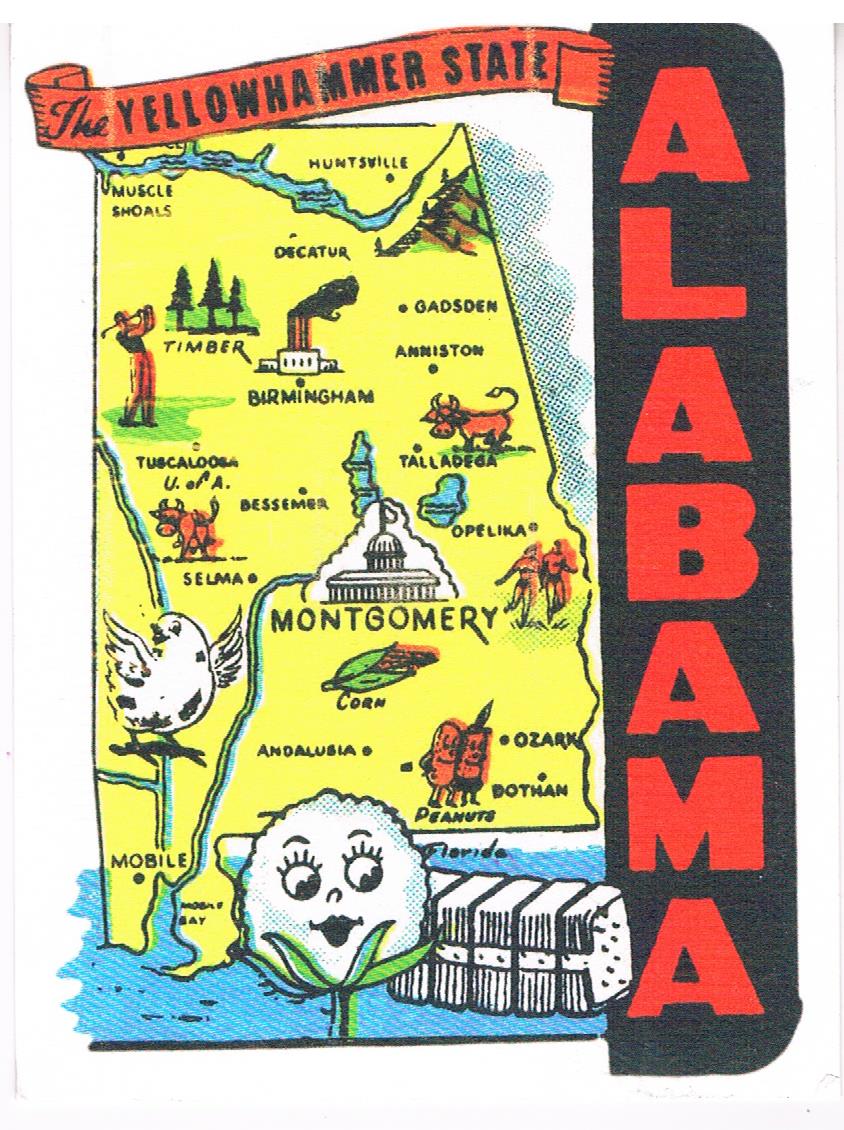This is a vintage-style poster for the state of Alabama. The left side of the image features a detailed, yellow-colored map highlighting key locations and landmarks within the state. Prominently marked cities and sites include Montgomery (situated centrally), Birmingham, Talladega, Opelika, Selma, Huntsville, Decatur, Gadsden, Anniston, Bessemer, Andalusia, Mobile, Ozark, and Bothan. The map also depicts important industries and natural features, such as rivers, timbers, and cotton fields. Illustrations accompany the textual information, showing trees, factories, animals, buildings, plants, a golf player, cows, corn, and the state bird. 

Above all these elements, at the top left corner, a red, curving ribbon banner reads "The Yellowhammer State" in black letters. On the right side of the image, a vertical black strip boldly features the word "Alabama" in red letters, written from top to bottom. The background and various details lend a rich and nostalgic touch, providing an inviting overview of Alabama’s characteristics and attractions.